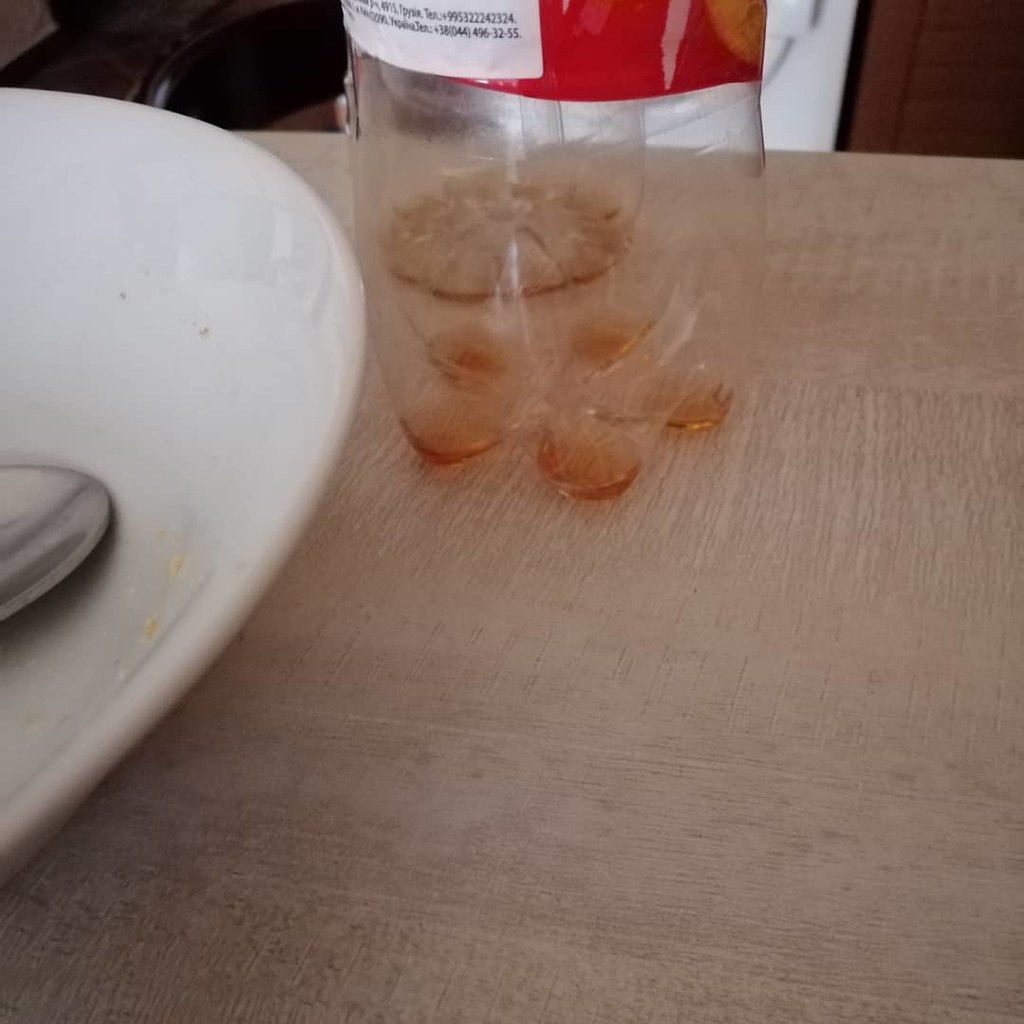The photograph captures the remnants of a meal on a worn Formica tabletop with a tan laminate veneer. Prominently, a plastic bottle with a red label, partly obscured, and a white label with unreadable text, sits on the table. The bottle contains a small amount of brown liquid and features the characteristic dented feet at its base, which allow it to sit flat even with a few droplets remaining. To the left, a large, partially visible white ceramic plate or bowl with a silver spoon peeking in from the edge shows a few scattered crumbs. The setting appears slightly cluttered, hinting at a casual meal, likely in a home given the surrounding details – such as a glimpse of a leather chair and what might be a brown door in the background.